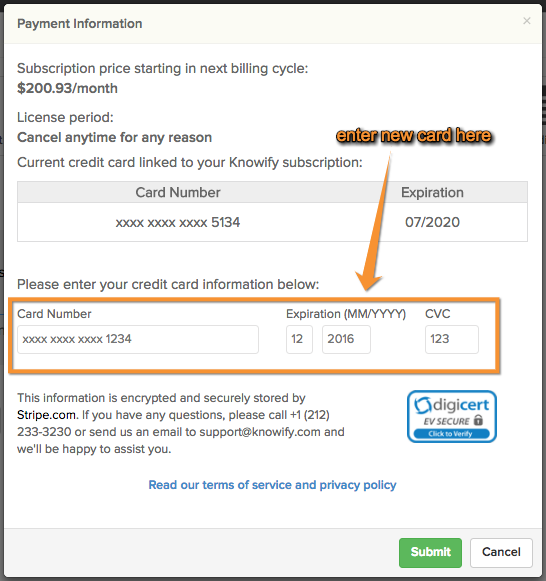The image displays a user-friendly payment information form for a subscription service. The form is organized neatly with key sections highlighted for ease of navigation. 

At the top, there is a heading titled "Payment Information" followed by a "Subscription" section. The subscription price is stated to be $200.93 per month, effective from the next billing cycle. Users are informed that the license period is flexible, allowing cancellation anytime for any reason.

Adjacent to the subscription details, a bold and prominent "Enter New Card Here" instruction is presented in a visually appealing coffee-colored brown font. A large arrow directs users downward to a dedicated section for entering card information.

Directly below the brown heading, there is a note mentioning the current credit card linked to the user's subscription, with placeholders for card number and expiration date. Users are prompted to enter their new credit card information within a brown-framed box, ensuring the section is clearly distinguishable.

The form is well-designed, providing all necessary details and instructions in a clear and aesthetically pleasing manner.